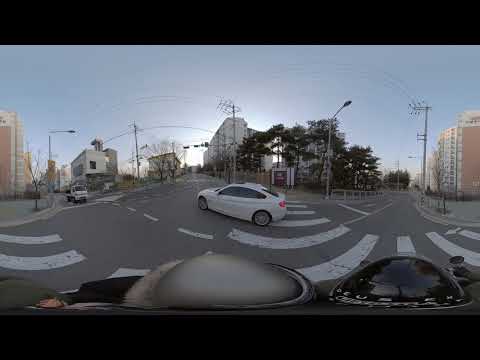The image captures a dynamic street scene viewed through a distorting lens, possibly from the handlebars of a motorcycle or the vantage point of a car. Central to the image is a white car situated in the middle of an intersection, with multiple roads branching from this point: one road to the right, two roads to the left of the midpoint. To the extreme left, another car or a truck appears to be waiting to cross. The scene is set against a backdrop of tall buildings partially obscured by trees. On the far left and far right of the image are multi-story buildings with a pinkish-beige hue. The sky above is a bright blue, illuminated by sunlight peeking through the buildings slightly to the left. Various elements such as crosswalks, light posts, and electrical posts add to the city ambiance. The photograph is distinctly urban, capturing the hustle of the city under the clear midday sky.